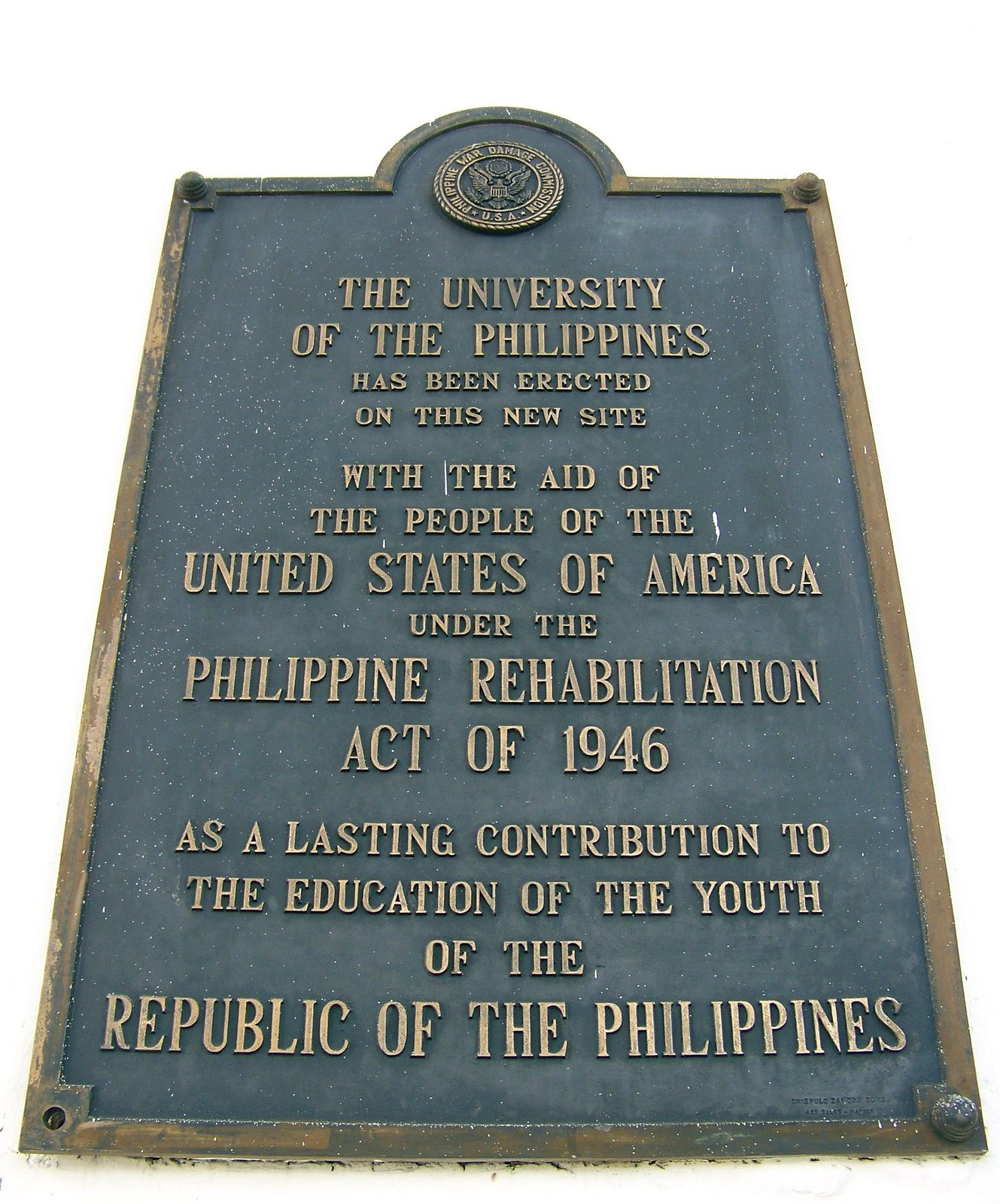This image depicts a commemorative plaque dedicated to the University of the Philippines, set against a white background with no surrounding context. The plaque is rectangular with a gold metallic border that appears tarnished, and it features a rounded top with the university's seal, depicting an eagle, situated in the arched center. The main body of the plaque is a charcoal-colored metallic surface with raised bronze or gold lettering that has a weathered appearance. Reading from a ground-level perspective, the inscription on the plaque states: “The University of the Philippines has been erected on this new site with the aid of the people of the United States of America, under the Philippine Rehabilitation Act of 1946, as a lasting contribution to the education of the youth of the Republic of the Philippines.” This plaque commemorates the historical act and symbolizes the enduring support for education in the Philippines.